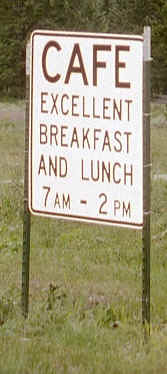In this image, we see a predominantly white, vertically rectangular sign that occupies most of the photo. At the top of the sign, the word "CAFE" is prominently displayed in bold black letters. Beneath it, the sign reads "Excellent breakfast and lunch" in successive lines. The hours of operation, "7 a.m. through 2 p.m.," are also noted. The sign is positioned on a patch of lush green grass, and in the background, there is a dense cluster of dark green trees. The sign itself measures approximately 4 to 5 inches in height.